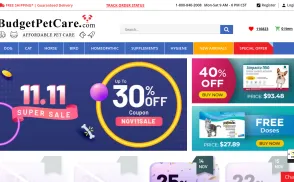BudgetPetCare.com is celebrating Valentine's Day with a sale. The image shows a cheerful white dog standing against a vibrant pink background sprinkled with confetti. To the right, text announces various discounts: "15% off", "40% off", and "25% off for Cat Month". Prices are also displayed, including "$93.48" and "$27.89" for free doses. Additionally, a prominent "Buy Now" button invites shoppers to take advantage of the offers. Some text remains too blurry to read.